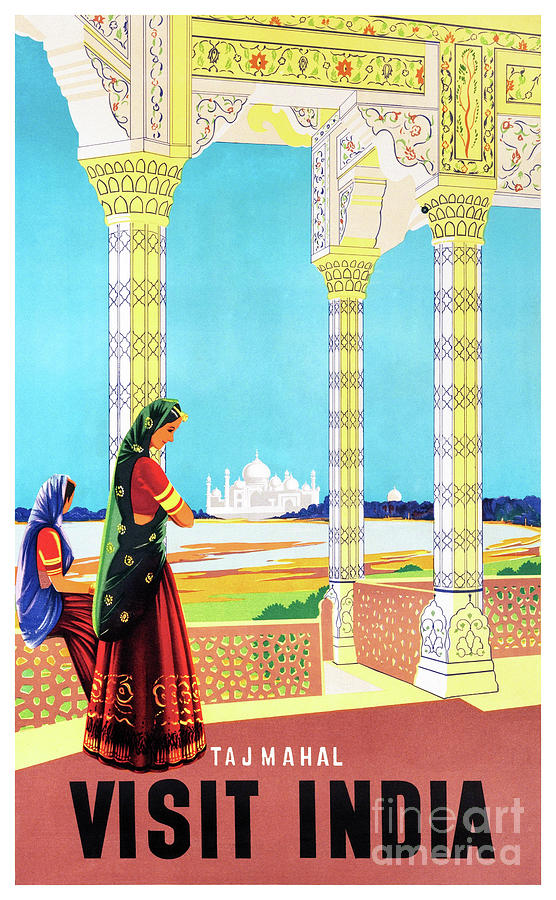This vertical, rectangular poster is a vibrant, cartoon-style drawing promoting travel to India. The bottom of the poster features a bold, promotional text: "Visit India" in large black letters. Above this, "Taj Mahal" is written in elegant white letters. The scene is set within an intricately decorated building with large, ornate pillars, adorned with yellow and red flowers and curves, and an equally elaborate horizontal element spanning across the top. In the background, framed by two of these pillars, stands the iconic, white Taj Mahal against a clear blue sky.

In the foreground, two Indian women are on the platform. The woman standing in front is fully visible, dressed in a red sari with yellow markings and a green robe featuring yellow patterns draped over her. She wears a red shirt that exposes a bit of her midriff and is detailed with a red and yellow band. Next to her, a second woman is seated, adorned in a red top with a gold border, a red skirt, and a blue headdress that extends down to her waist. The scene is completed by an orange fence near the base of the columns, contributing to the rich, colorful composition. The watermark at the bottom reads "Fine Art America."